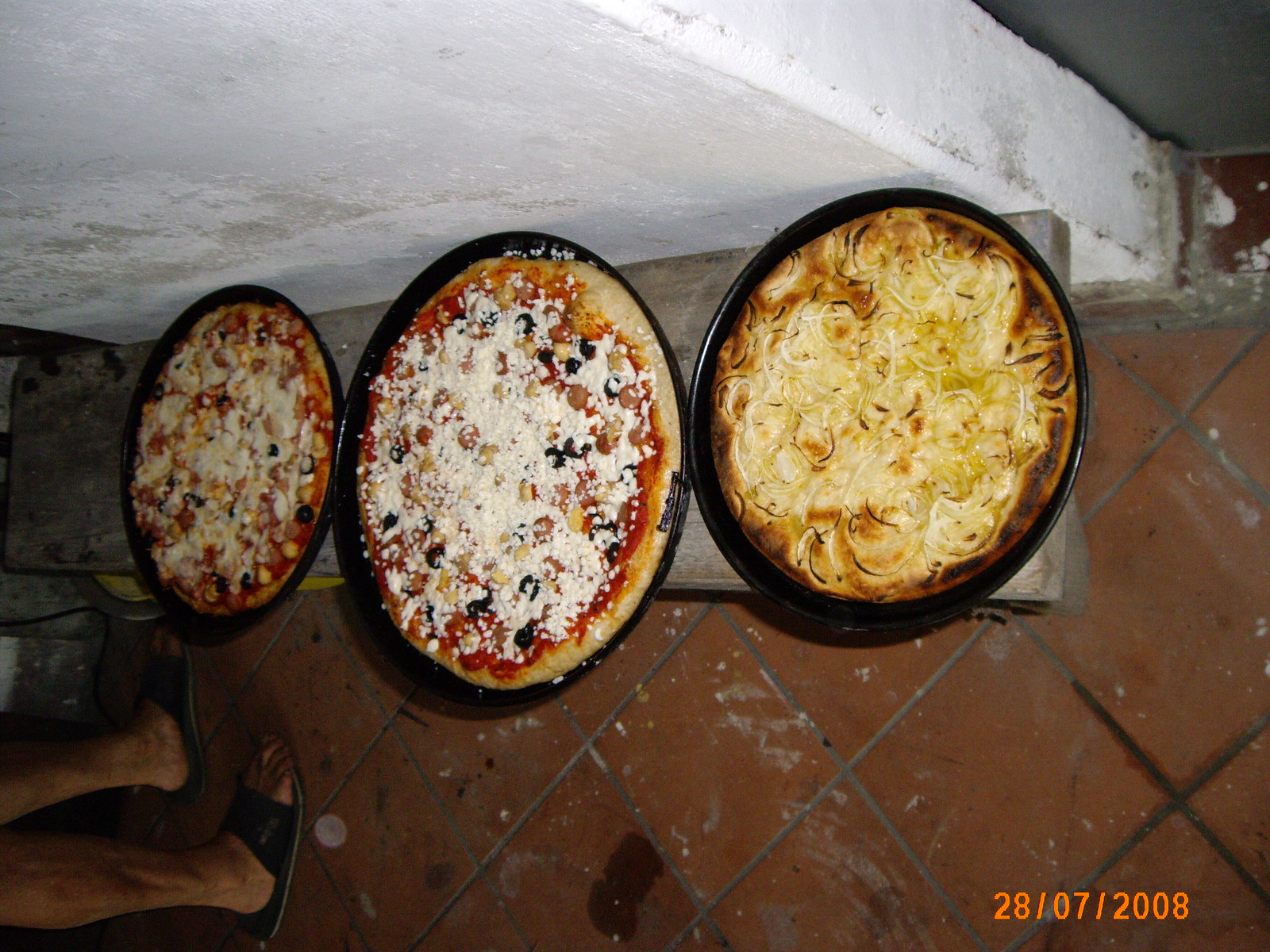The photograph, dated 28 July 2008, captures a top-down view of three pan pizzas placed on a low wooden bench or shelf, positioned about a foot off the floor. The pizzas are displayed in black pans and vary in size and toppings: the middle one being the largest, flanked by two medium-sized ones. The one on the right appears to be slightly burnt around the edges and is topped with white cheese and onions. The middle pizza is adorned with tomato paste, olives, various cheeses including feta, and possibly mozzarella, while the left pizza has tomato sauce, cheese, and a mix of toppings like mushrooms, corn, and possibly sausages.

The scene is set in a very dirty, industrial-looking kitchen with a grubby brown or red tile floor stained with paint splatters and dust. A pair of legs wearing black slide sandals is visible in the bottom left corner, suggesting the presence of someone in the space. The background features a concrete or white wall, against which the shelf is mounted. The overall impression is one of a casual, perhaps impromptu setting, possibly indicative of a personal kitchen or a makeshift cooking area.